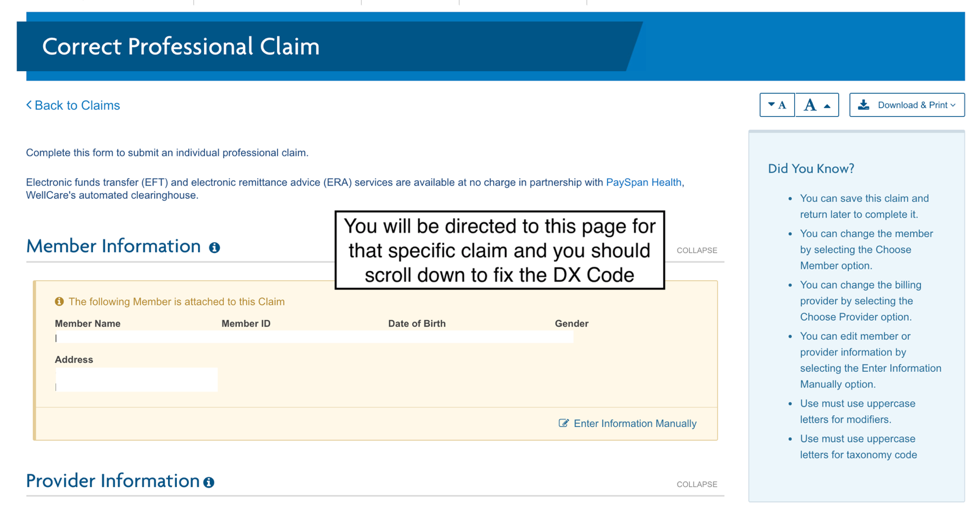The image depicts a detailed interface for submitting a professional claim. 

At the top of the screen, there's a blue-bordered header titled "Correct Professional Claim." Below it, on the left side, is a "Back to Claims" button. The main body of the interface contains several informative sections.

Starting with instructions, the first description reads: "Complete this form to submit an individualized professional claim." Immediately below, a second instruction specifies that electronic funds transfer (EFT) and electronic remittance advice (ERA) services are offered for free in partnership with Payspan Health, under WellCare's automated clearinghouse.

Under these instructions, there is a "Member Information" section marked by an 'i' icon. A smaller, overlapping box prompts users, stating: "You will be directed to this page for that specific claim. Scroll down to fix the DX code."

Underneath the "Member Information," a yellowish box indicates the following member details attached to the claim: "Member Name, Member ID, Date of Birth, and Gender." Currently, these fields are blank. At the bottom, there's an "Address" field with an "enter information manually" option for editing.

Further down is a "Provider Information" section highlighted in blue, though it displays no additional content at the moment.

On the right side, there are options for downloading and printing the form, distinguished by an 'A' and a larger 'A' indicating different capitalization options. 

A blue column titled "Did You Know?" provides six tips for users. It explains that users can save the claim and return to complete it later, change the member of voice, choose member options, modify billing, and access six specific tasks through clickable hyperlinks.